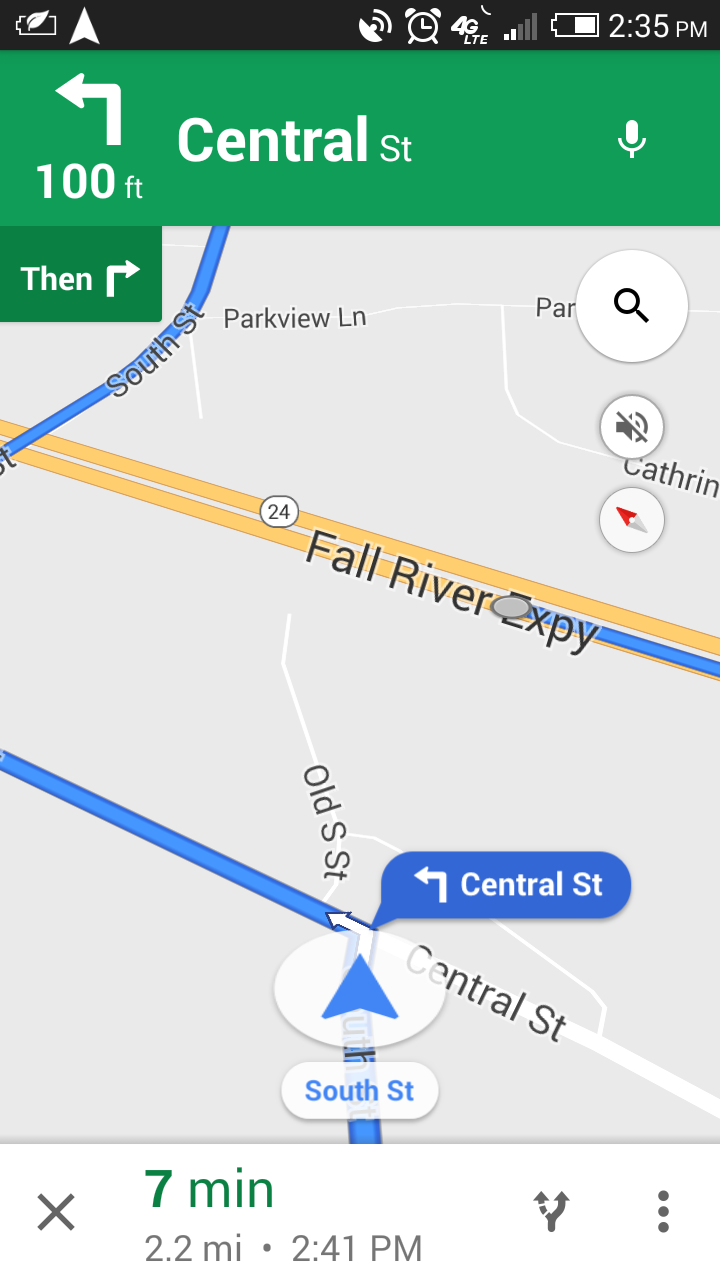The screenshot captured from a smartphone displays Google Maps directions. Evident from the phone icons at the top, including various notifications, GPS signals, the battery indicator, and the time marked at 2:35 p.m., it is clear that this is a mobile device. The main portion of the screenshot shows a segment of the map with crucial navigational details. The map has a predominantly white background with blue lines indicating the route to be followed. Notably, the driver is instructed to turn left onto Central Street in 100 feet.

A light yellow line on the map marks the Fall River Expressway. The top of the screenshot features directions against a green background with white text, ensuring clear visibility. At the bottom, the estimated time of travel is prominently displayed in green as "7 minutes," with a distance of "2.2 miles" written in black. Adjacent to these details is the expected time of arrival indicated as "2:41 p.m."